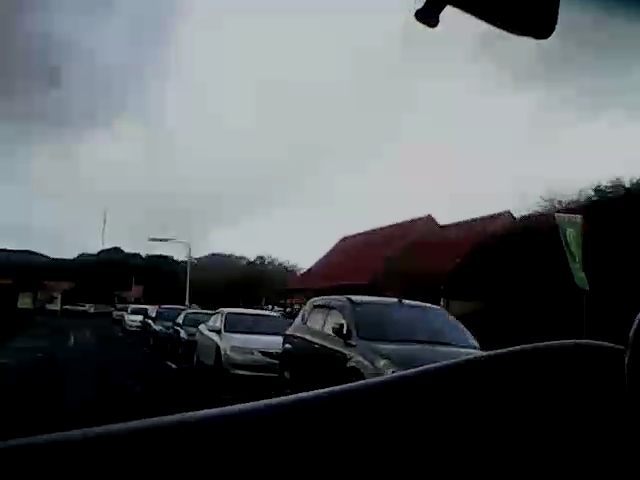A lineup of various cars is parked in front of a prominent red building, which features a red roof. Attached to the building, a green sign resembling a flag hangs from the side. The vehicles seem to be stationary, potentially waiting for an event or parked temporarily. A traffic divider is in place to prevent further vehicle movement. A large street light indicates the outdoor setting, which includes additional buildings and trees visible in the distance. The sky above is overcast and grey, suggesting imminent rainfall.